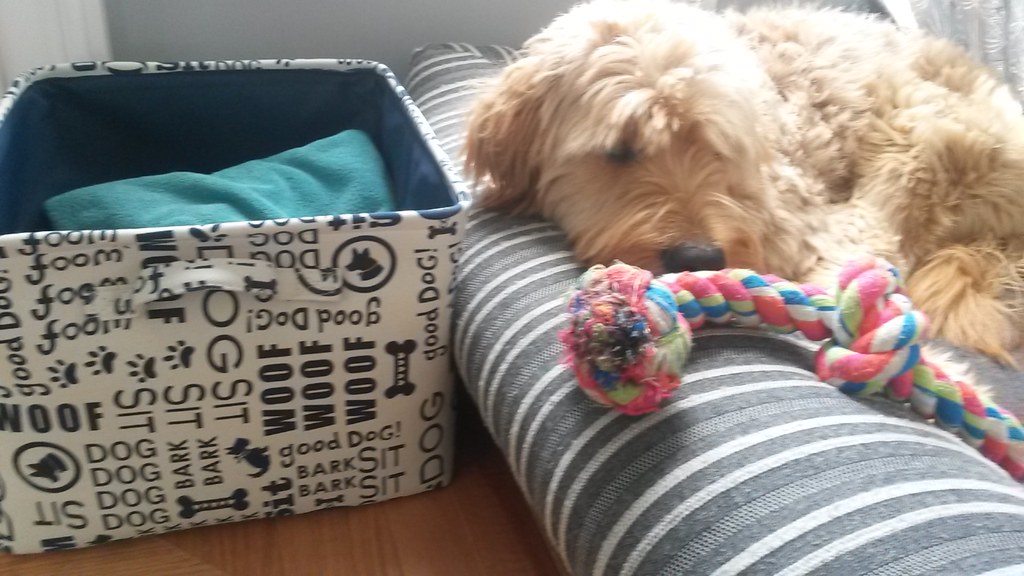This detailed photograph captures a close-up view of a charming, medium-sized golden doodle with a sandy coat of fur, resting peacefully on a couch. The dog occupies the right half of the image, lounging comfortably on a grey and white striped dog bed. One eye is partially open and the other obscured by its fluffy hair, giving it a slightly somber expression as it snuggles near a colorful dog rope toy composed of red, blue, green, and white threads, which is positioned near its nose.

To the left of the golden doodle, there's a fabric storage box adorned with playful dog-related phrases such as "woof woof woof," "sit sit sit," "dog dog dog," and "good dog." The top of this cubicle is open, revealing a simple, folded blue blanket inside. The setup, partially on a wooden table, suggests a cozy, well-loved space for the furry companion. The overall feel of the scene is one of domestic tranquility and affection, centered on the mellow presence of the dog.